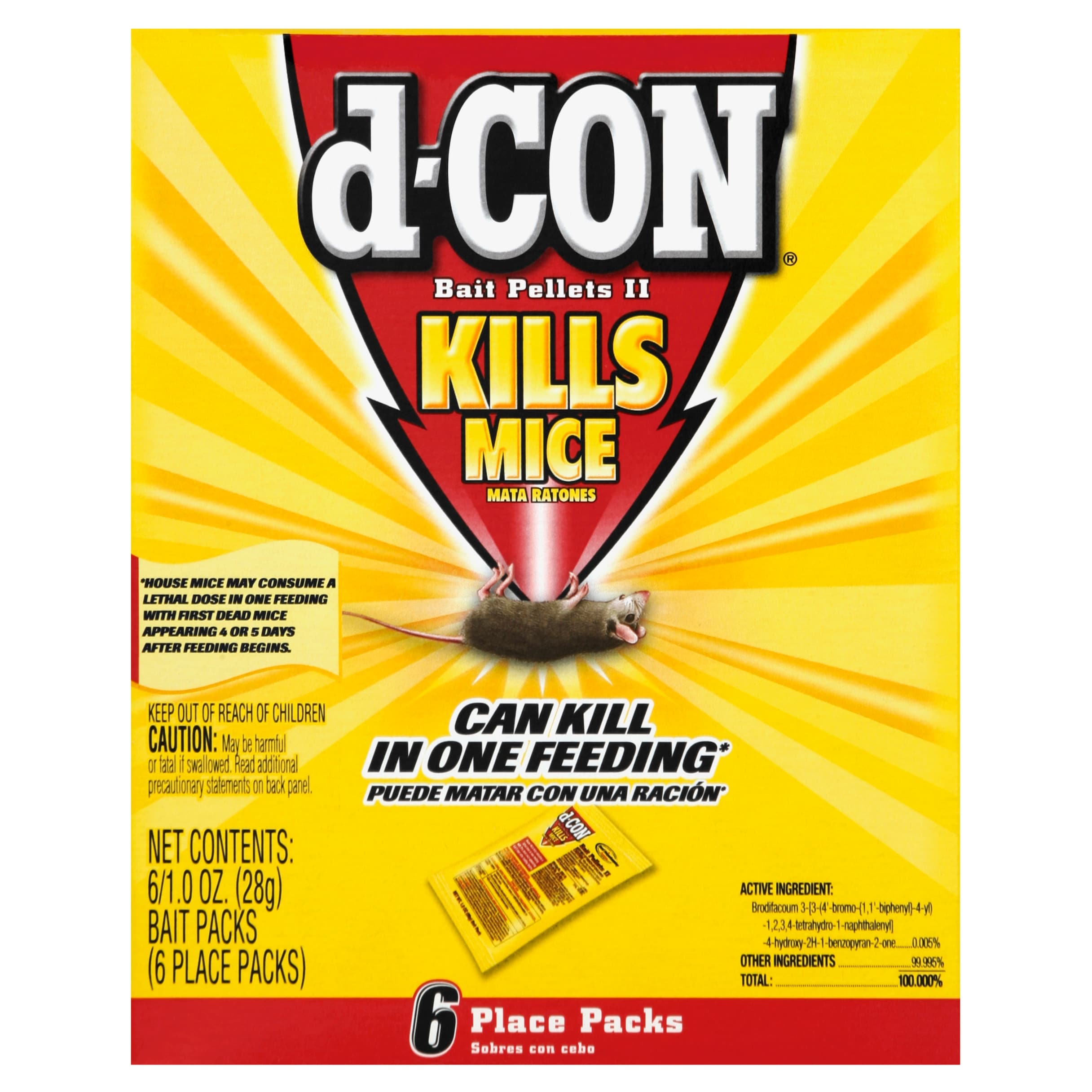The image is a vertical color photograph showcasing the front of a rectangular box of Decon Bait Pellets 2. The background is predominantly yellow, with some red accents. The top of the box prominently features "Decon" in large white letters, followed by "Bait Pellets 2" and "Kills Mice" in smaller yellow text, along with a Spanish translation "mata ratones." Below this, there is a detailed, realistic drawing of a dead mouse laying on its back with its feet sticking up, emphasizing the product's effectiveness. The box touts that the bait can "kill in one feeding," and specifies, "house mice may consume a lethal dose in one feeding, with first dead mice appearing four or five days after feeding begins." Further down, it indicates that the package contains six place packs and provides a picture of what the individual packets look like. On the right-hand side, there are details about the active ingredients and other components, accompanied by a cautionary message to keep the product out of reach of children and another warning to read additional precautionary statements on the back panel. The bottom left-hand corner includes additional information about the net contents and weight, and the bottom border of the box is highlighted in red, reiterating "six place packs" in bold font.